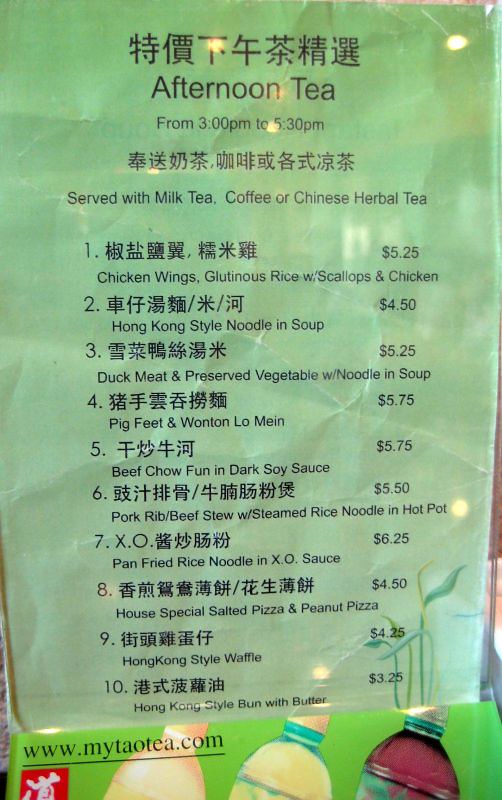A photograph showcases a bilingual menu featuring both Chinese and English text. The English section headlines "Afternoon Tea from 3pm to 5:30pm," inviting patrons to enjoy their tea accompanied by either milk tea, coffee, or Chinese herbal tea. Below the header, a list of enticing menu items is provided:

1. Chicken wings, glutinous rice with scallops and chicken
2. Hong Kong style noodle in soup
3. Duck meat and preserved vegetables with noodle in soup
4. Pig feet and wonton lo mein
5. Beef chow fun in dark soy sauce
6. Pork rib beef stew with steamed rice noodle in hot pot
7. Pan fried rice noodle in XO sauce
8. House special salted pizza and peanut pizza
9. Hong Kong style waffle
10. Hong Kong style bun with butter

The menu concludes with the establishment’s website: www.mytaotea.com.